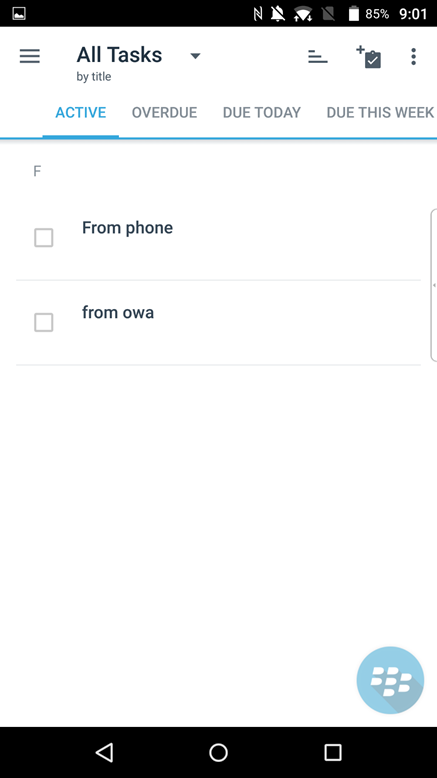This screenshot from a smartphone displays a richly detailed user interface. At the top, the status bar shows several icons: a gallery symbol, active Wi-Fi notifications, an SD card icon, and a battery life indicator at 85%. The current time is 9:01 AM. 

Beneath this status bar, there is a list titled "All Tasks by Title" categorizing tasks under several statuses: "Active," "Overdue," "Due Today," "Due This Week." These categories help keep the user organized and aware of pending responsibilities. 

Additionally, there are labels indicating the source of some tasks, specifically "From Phone" and "From OWA" (Outlook Web Access).

At the bottom of the screen, the navigation bar contains three standard Android navigation buttons: a 'Back' button, a 'Home' button, and a 'Tab' button. There is also a blue dial pad with seven white dots, adding an interactive element for task or number input.

In summary, this screenshot presents a well-organized and interactive smartphone interface designed to keep the user informed and efficient.